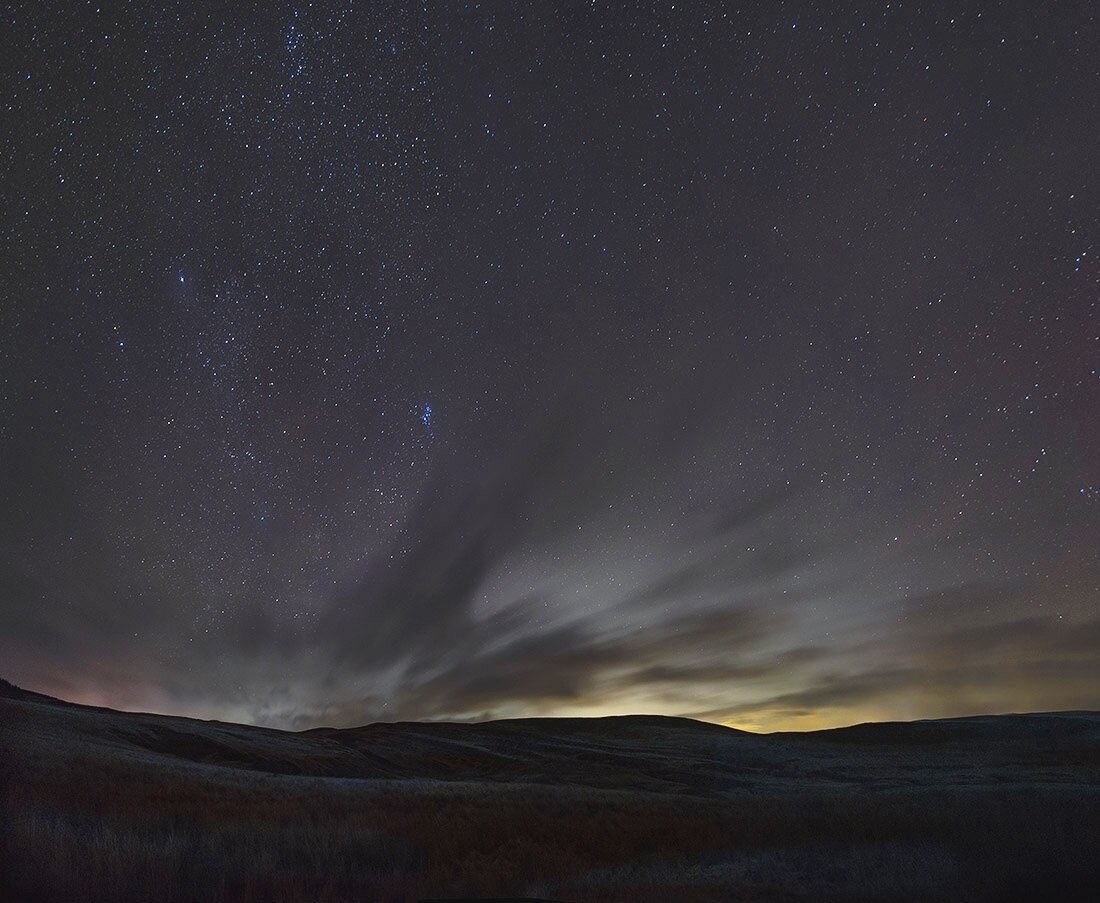This photograph captures a captivating outdoor natural setting during the late evening or nighttime. The scene features an uneven, grassy terrain at the bottom, with the grass appearing dark, possibly brown or orange in color. Above this, dark mountains create a stark silhouette against the sky. The sky itself is a mesmerizing blend of dark hues, ranging from charcoal gray to deep purple. It is speckled with countless stars, some of which shine brightly like white and bluish fairy dust, lending a whimsical aura to the scene. Dark clouds, resembling streaks in motion, hover near the horizon where there is a faint hint of a yellow gradient, suggesting the remnants of sunset or the first light of dawn. This interplay of celestial and terrestrial elements conveys a serene and peaceful atmosphere.